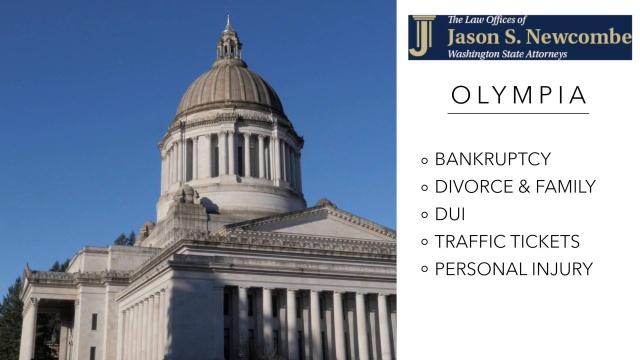This advertisement for the Law Offices of Jason S. Newcomb, Washington State Attorneys, features an exterior photograph of the majestic white and gray rotunda of a state capitol building, set against a bright blue, cloudless sky. The building's architectural details, including its grand pillars and towering dome, evoke a sense of authority and stability. Positioned to the left of the image are treetops that add a touch of greenery to the scene. To the right of the photograph is the firm's logo and text in a sleek silver-brown color, listing "Bankruptcy, Divorce and Family, DUI, Traffic Tickets, and Personal Injury" as their areas of practice. Below the firm's name and logo is the location "Olympia." The professional and clean design of the ad emphasizes the firm's dedication and specialization in their legal services, set against a crisp white background.